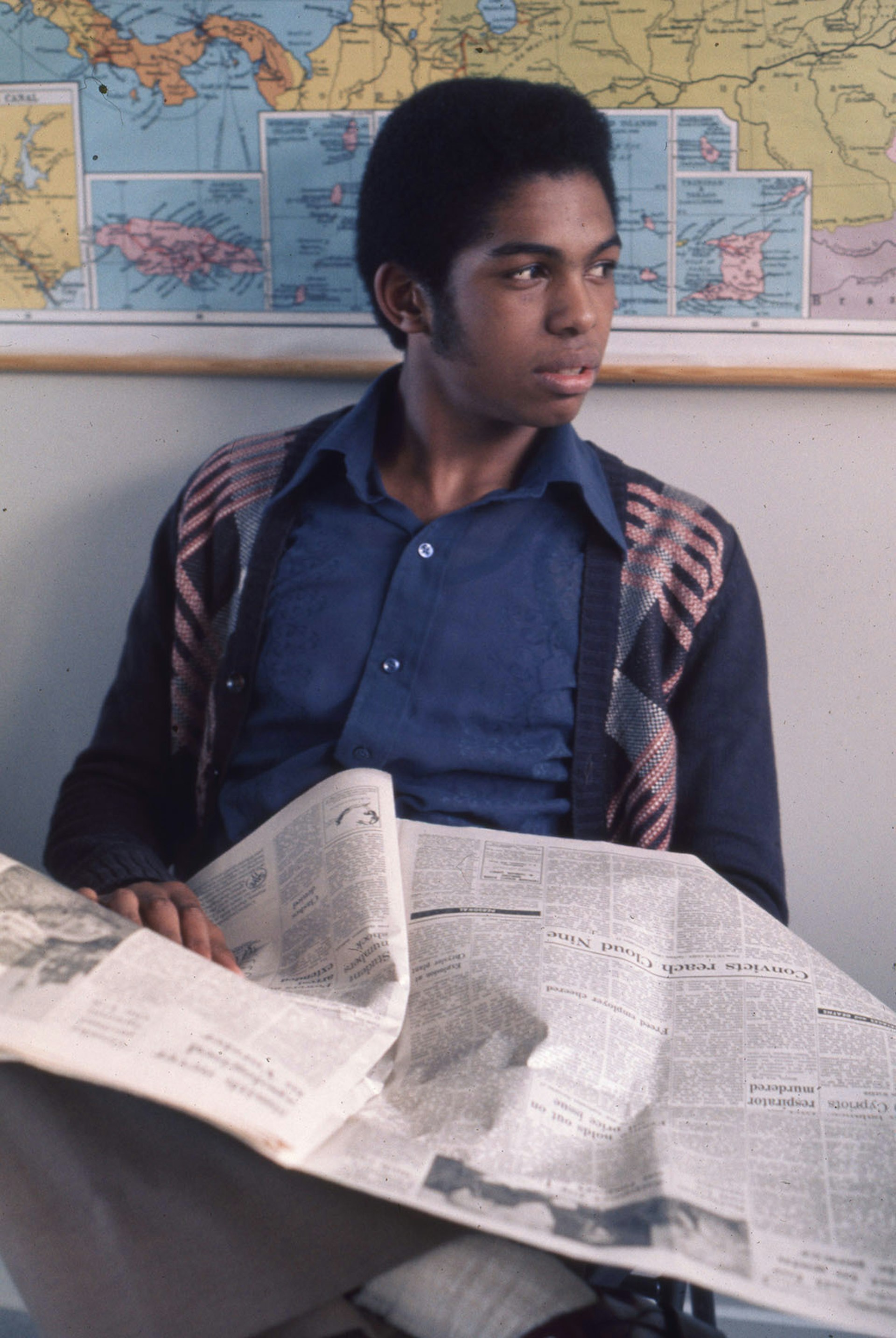This photograph captures a young black man with brown skin, dressed in a blue button-down shirt layered under a dark blue sweater with pink stripes. He sports a flat top haircut with noticeable mutton chop sideburns. Sitting with his legs crossed on a chair, he holds a crinkled-up newspaper in his lap and gazes thoughtfully off to the right. Behind him is a wall adorned with a framed colored map, showing indistinguishable land masses, possibly depicting South America with its notable traits like the Panama Canal. The overall setting, including the young man's attire and the photographic style, suggests a nostalgic feel reminiscent of the late 1980s or early 1990s.